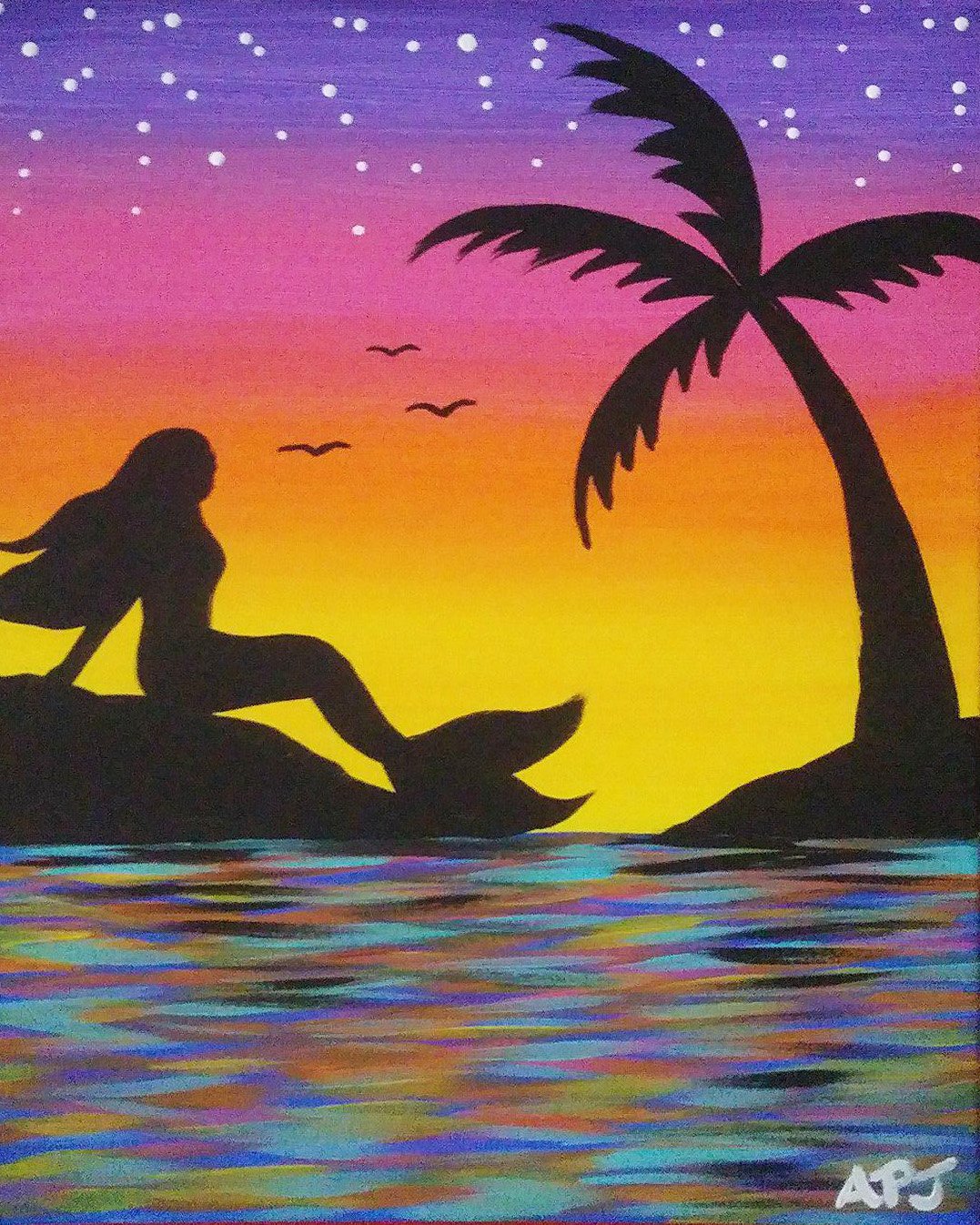This painting captures a vivid and colorful seascape at sundown. The background features a dramatic sky that transitions from a deep purple at the top, sprinkled with white stars, to hues of pink, orange, and finally yellow near the horizon. The vibrant watercolor extends into the ocean below, reflecting shades of blue, teal, black, yellow, and red. On the left side of the composition, a black silhouette of a mermaid with flowing hair and a visible tail sits on a small rocky landform, her arms resting behind her. Meanwhile, on the right side, there is another silhouetted piece of land adorned with a palm tree. Between these two landforms, three V-shaped birds are seen flying distantly across the colorful sky. The painting is signed at the bottom right corner with the initials "APJ."